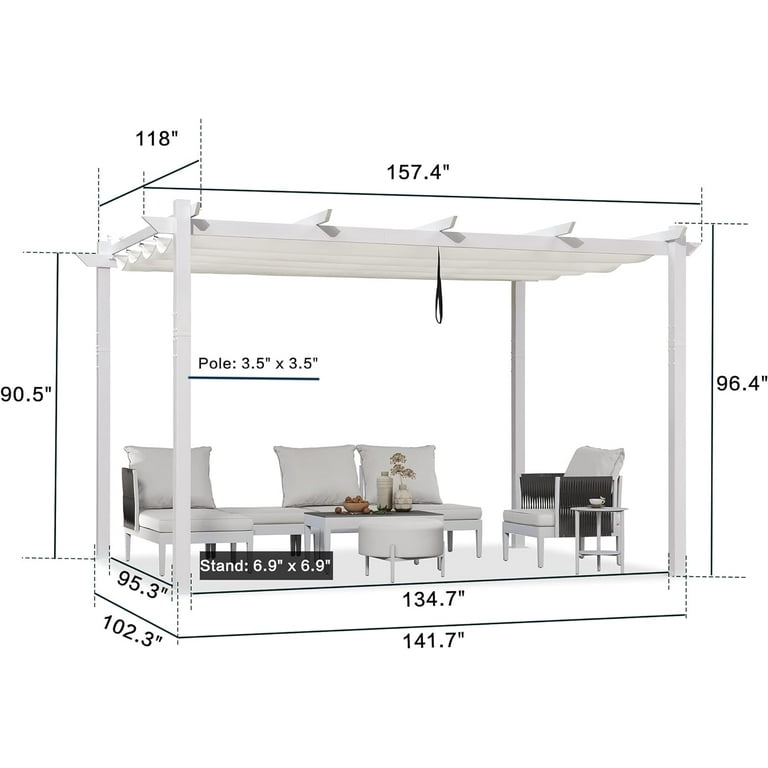This image shows a detailed diagram of a white pergola with specific measurements displayed. The pergola, open on all sides and covered by a drooping white beam ceiling, measures 157.4 inches on top, with the height of the supports up to the ceiling being 96.4 inches and 90.5 inches to the shorter roof. The width between the supports is 134.7 inches in the front and 95.3 inches on the side. The structure stands on four legs.

Inside the pergola, there is a harmonious arrangement of white patio furniture. On the left side, there is a comfortable white chaise lounge with a fluffy white cushion. To its right is a white loveseat adorned with two attached cushions and a small round white stool. Adjacent to the loveseat is a coffee table with a black top holding two white vases (one with a brown plant) and a brown bowl with round objects. Further to the right, there is a white side chair with black armrests and beside it, a small tall white side table with a white mug. In addition, there is a white side chair, and a small round table completes the setting. Dominating the center top of the pergola, a black strap hangs down. The seamless white background enhances the sophisticated and clean aesthetic of the image, making it suitable for a catalog or website depiction.